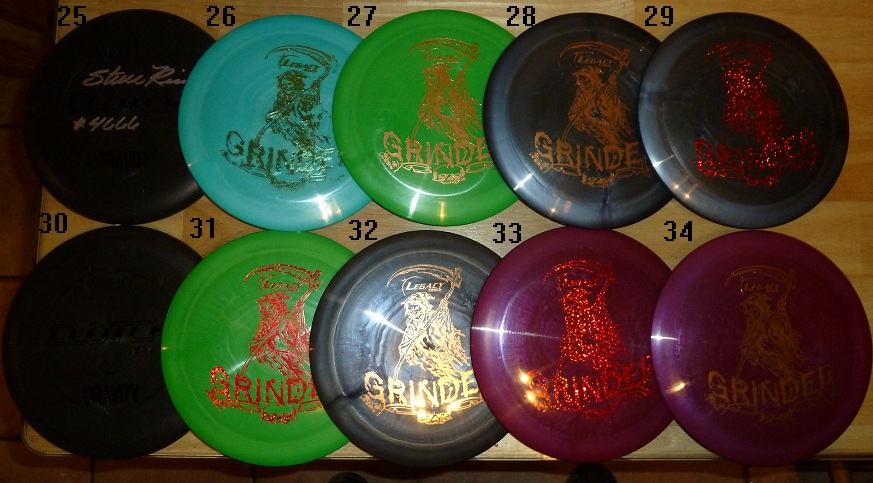This photograph captures a neatly arranged display of ten frisbees, commonly used for disc golf, set on a light-colored wooden surface that transitions to a darker brown background on the left with some visible holes. The frisbees are positioned in two rows of five, with small black numbers indicating their sequence from 25 to 34, placed just above and to the left of each disc. In the top row, the frisbees are colored black, blue, green, black, and black from left to right, and in the bottom row, they are dark green, black, burgundy, burgundy, and black. Each frisbee, except for the first two black ones on the top left, features the brand name "Grinder" and an image of a Grim Reaper in a metallic hue. Notably, one of the frisbees displays a signature and the number 4666, adding a unique touch to this collection of vibrant and meticulously presented sporting equipment.